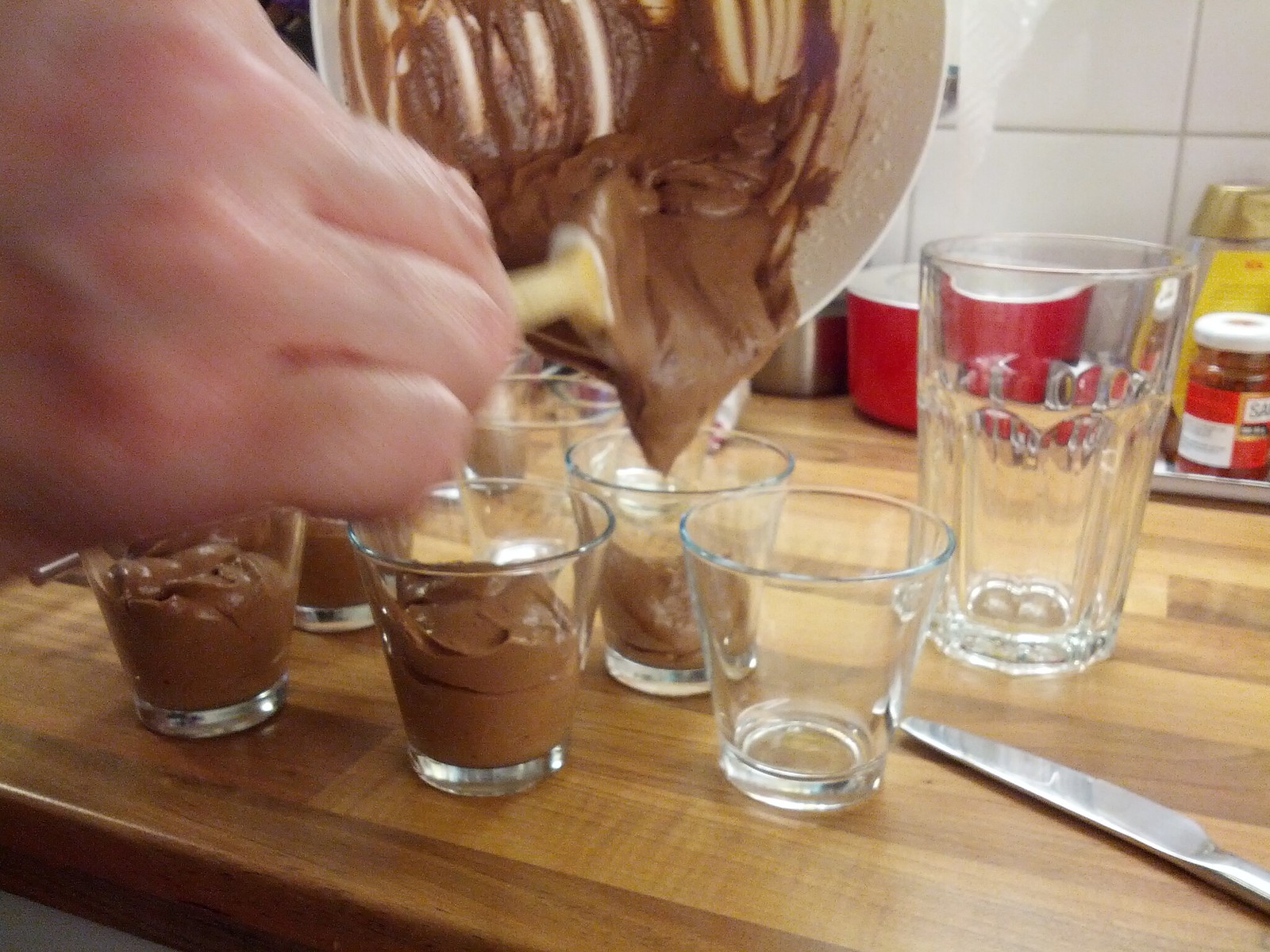In this close-up action shot, a Caucasian hand, partially visible from the upper right corner, is prominently foregrounded as it uses a yellow spatula to scoop chocolate mousse from a white bowl. The bowl is tilted sideways, revealing the rich, brown mousse being carefully poured into small, clear tumblers, resembling miniature drinking glasses that are slightly wider than standard shot glasses. Three of these glasses are already full, a fourth is being filled, and a fifth remains empty, lined up on a butcher block-colored countertop. In the background, the kitchen setting includes a blurred view of white tiled backsplash, a red empty bowl, a silver tray possibly containing unidentifiable ingredients, and a larger empty drinking glass. A silver butter knife rests on the countertop near the glass tumblers, completing the scene rich with culinary activity.